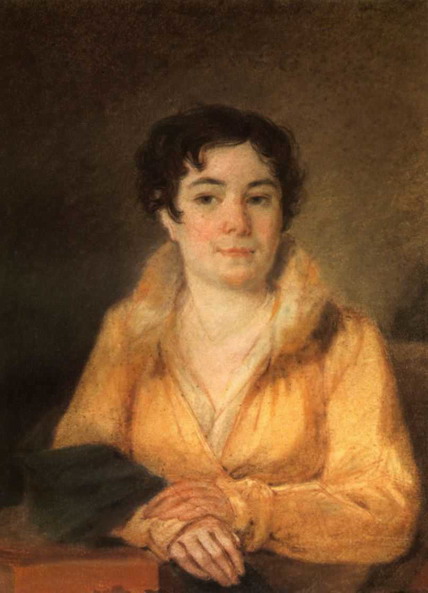This detailed portrait of a woman features her with short, semi-wavy dark brown hair, which falls to mid-ear length. Her fair skin showcases rosy cheeks, dark eyes, and full, dark eyebrows. The woman’s lips are painted a soft pink, and she is looking slightly to the right with a gentle, closed mouth expression. She is dressed in a pale yellow-orange dress with long sleeves and a v-neck, which has the collar turned up. Underneath, a hint of a light pink garment can be seen. A piece of dark gray or charcoal fabric is wrapped around her right elbow. Her hands are elegantly placed in front of her, with her left hand resting on her right wrist. The right elbow is supported by a small, square brown object, possibly a table. The background transitions from a soft brown to darker brown shades, imparting a warm and fuzzy feel to the image, as if created with soft brush strokes to give it an overall gentle and slightly hazy texture.